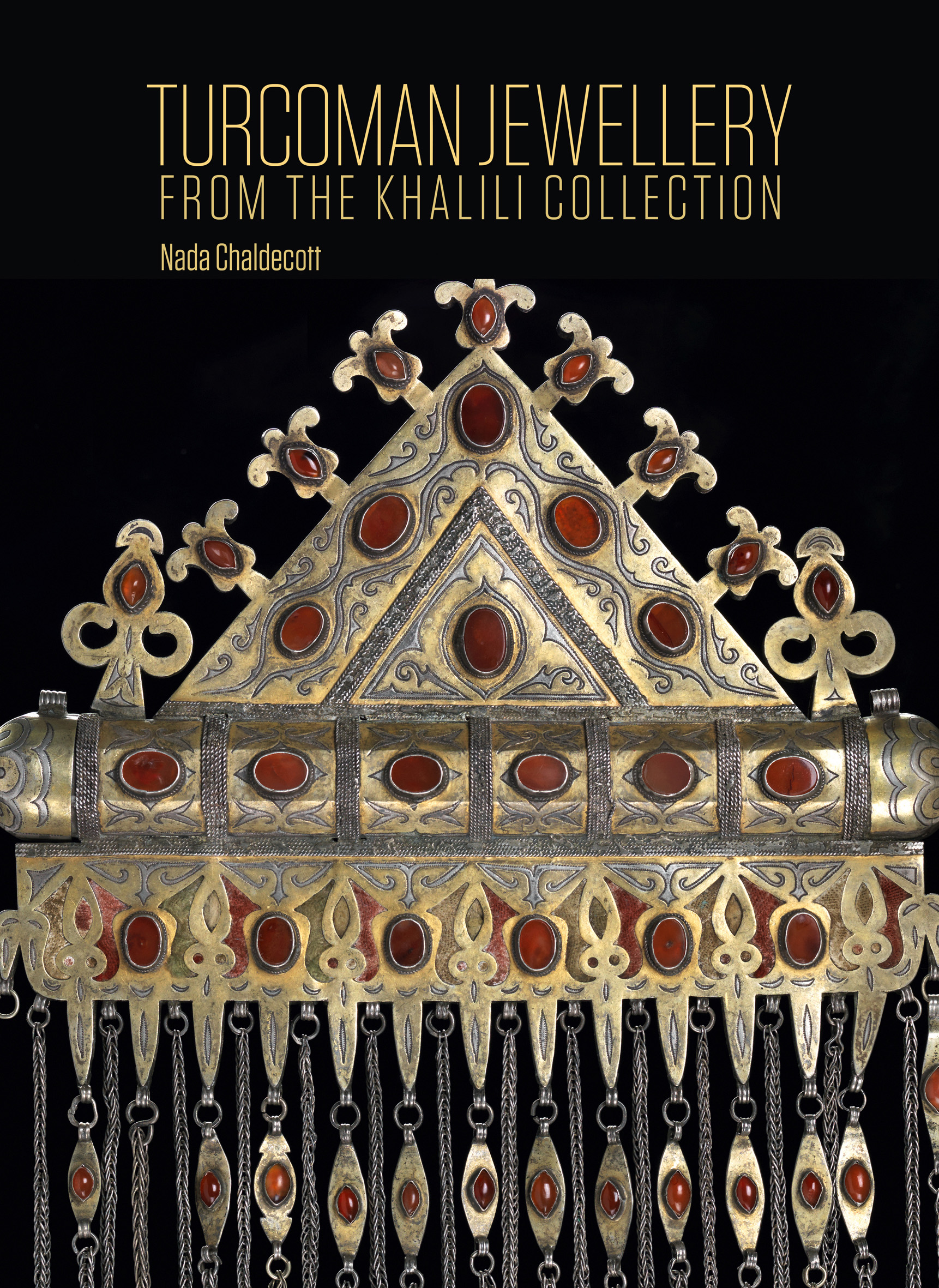This image, oriented in portrait style, features a black background with prominent yellow uppercase letters at the top that read "Turcoman Jewelry from the Khalili Collection," followed by smaller text stating "Nada Chaldecott." The central visual element is an intricate piece of jewelry, potentially a headpiece or a crown, characterized by a large central triangle adorned with red ovals resembling rubies. The triangle is bordered by intricate, flower-shaped designs, each also embellished with similar red ovals. This elaborate piece primarily sports a brassy hue, suggesting a metallic composition. Beneath the main triangle and flower designs, there are two horizontal bands also studded with red ovals, indicative of rubies. From these bands, numerous brass pieces and chains dangle, adding an ornate and dangly aspect to the overall design.